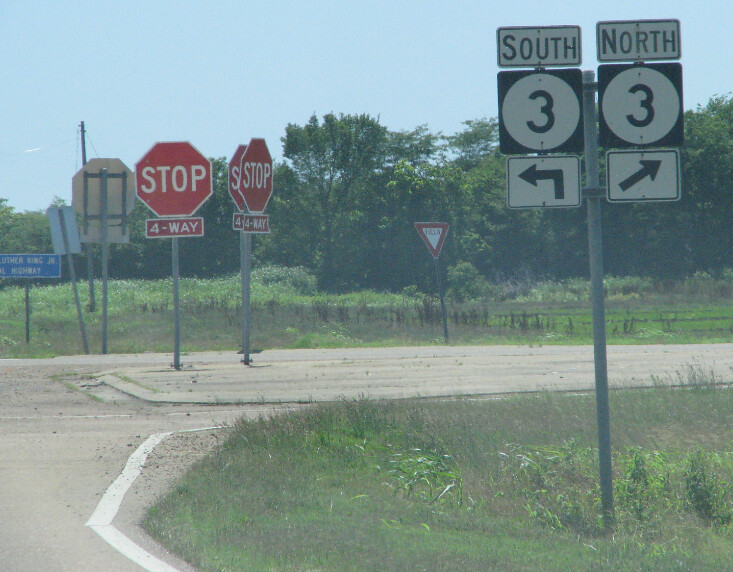This is a detailed photograph of an intersection likely located in Mississippi or Alabama, characterized by its unkempt, country-road appearance. The intersection appears cluttered with an unusual number of stop signs—four in total—clustered in the median, all visible within the scene. Additionally, there is a yield sign placed farther off. The signage indicates that turning left leads to South Highway 3, while turning right directs you to North Highway 3, with corresponding arrows and the highway number encapsulated in white circles. The median itself is a greyish stone, intersecting lanes travelling in opposite directions.

In the foreground, there is grass leading up to the intersection, which features a road crossing perpendicularly. Beyond the intersection, a sprawling meadow and bayou-like trees stretch into the distance, reinforcing the Southern, possibly rural, setting. A blue sign marks this area as part of the Martin Luther King Jr. Memorial Highway. The scene is quite serene and empty, with no vehicles present, set against a cloudless blue sky. A lone telephone pole can be seen faintly in the far distance, completing the pastoral landscape.